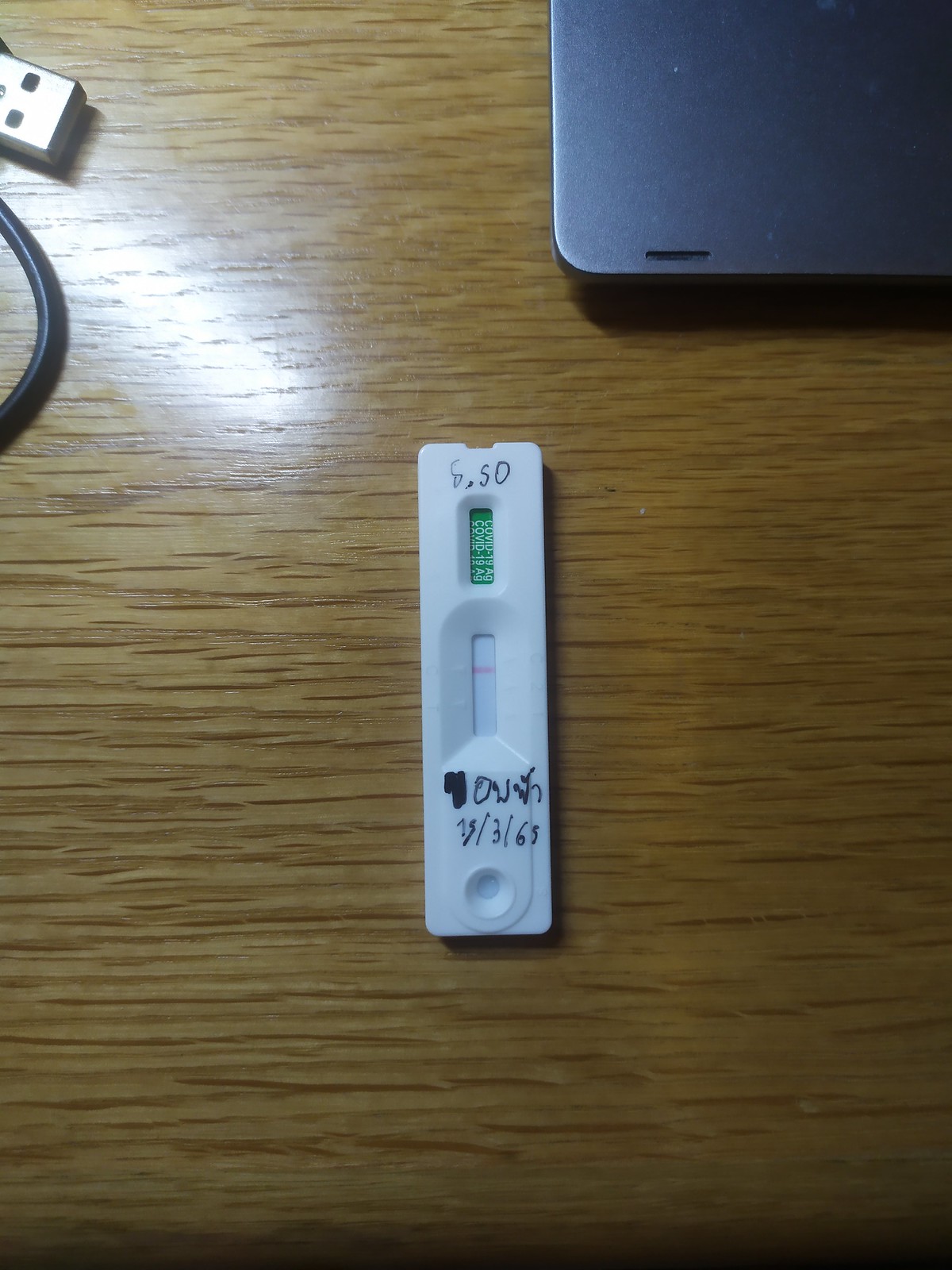This photograph, taken on a table, presents a detailed view of a testing kit at its center. In the background, on the top left, a segment of a black USB 2.0 cable is visible, while the top right shows a portion of a laptop, possibly where you would rest your wrists while typing.

The primary focus of the image is the testing kit itself. This white, rectangular device, roughly the size of a USB stick, features two distinct screens. The first, situated towards the top, has a green, digital appearance. Below it is the main testing screen, common in diagnostic kits, which is primarily white with a single red bar at the top, indicating a result. 

Beneath this main screen is some text, not written in English, and a sequence of numbers, "25365", which may represent specific test readings or codes. An indentation or small circle divot likely serves as the sample collection area for saliva, blood, or another biological sample. Additionally, there's text at the top of the kit, possibly indicating a time or reading, which appears to be either "5.50" or "6.50".

Overall, the image captures a well-used, manually labeled testing kit amidst a few peripheral electronic items, suggesting a casual or home-testing environment.